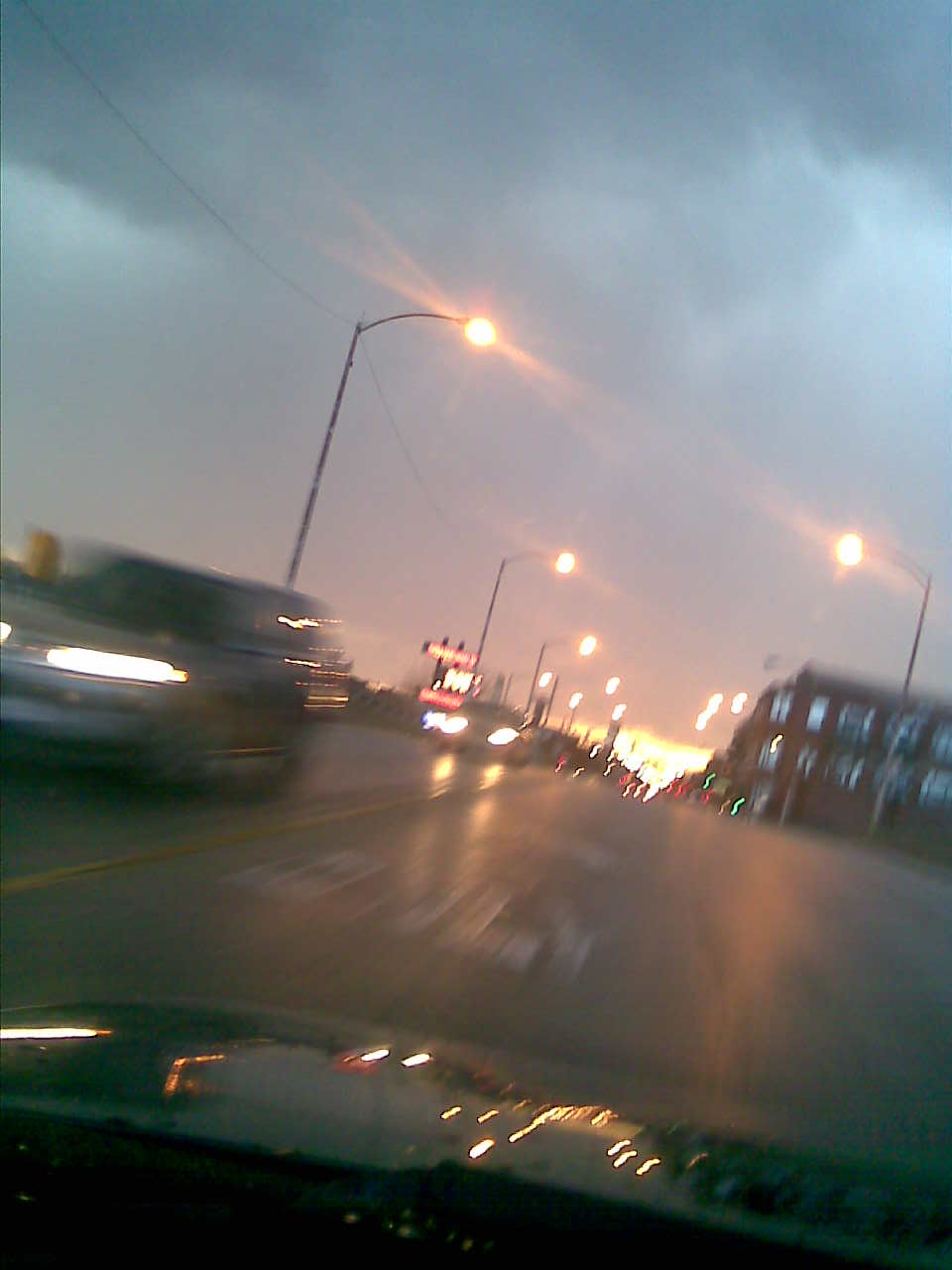The image captures a dynamic scene from within a moving car, either during the early morning or early evening, as evidenced by the low, soft lighting indicative of the sun poised just below the horizon. The sky is laden with heavy cloud coverage, casting a subdued light over the area, while numerous street lights remain illuminated, highlighting the transition between day and night. In the background, a prominent building stands tall, accompanied by vibrant neon signs in white and red, hinting that the setting is likely a bustling downtown or city area. To the right, another car speeds past, contributing to the scene's sense of motion, which is further emphasized by the overall slight blur of the image.